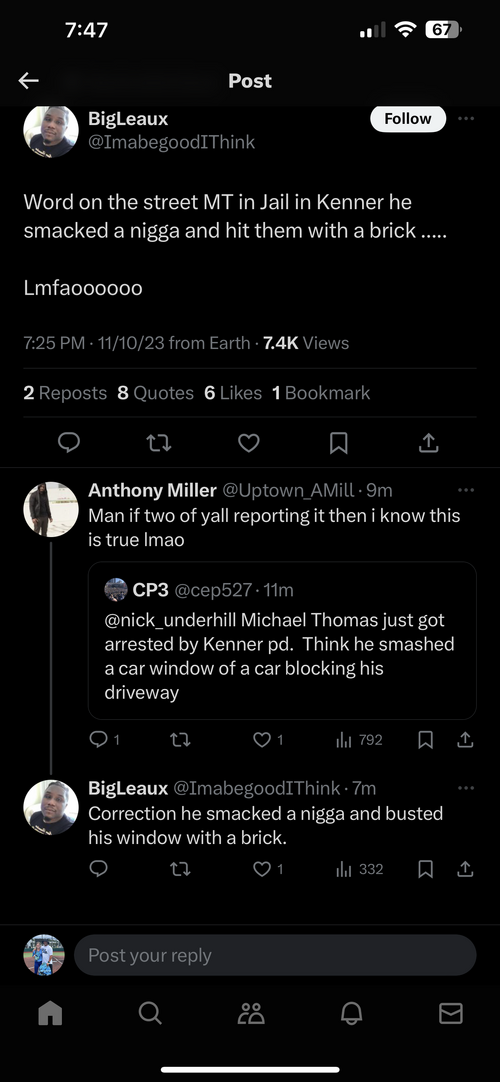Image Description for Social Media Post:

The image captures a typical mobile phone screenshot with a black background. At the top, a notification bar indicates a battery level of 67%, with two bars of signal strength and the time displayed as 7:47 PM. The word "Post" appears at the very top, suggesting the platform used.

The main content is a purported social media post by a user named "Big Leaux," featuring a profile picture of an African American man and a white "Follow" button next to his username. The post's text reads: "Word on the street MT in jail in Kenner. He smacked a nigga and he'll hit them with a brick. L M F A O O O O."

Below the post, engagement metrics reveal there are 2 reposts, 8 quotes, 6 likes, and 1 bookmark. In the comments section, one user states, "Man if two of y'all reporting it then I know this is true," while another comment reads, "Thomas just got arrested by Kenner PD. Think he smashed a car window of a car blocking his driveway." The original poster, Big Leaux, responds with a correction: "Correction he smacked a nigga and busted his window with a brick."

At the bottom of the screen, there is a text field labeled "Post your reply" for adding new comments, accompanied by the standard phone icons for navigation.